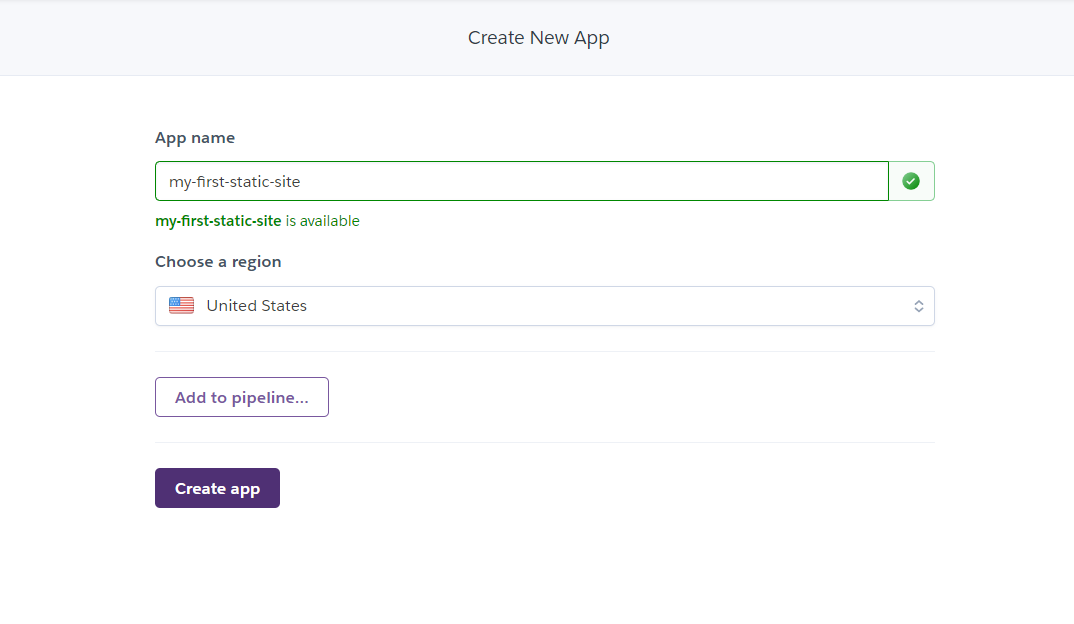The image showcases a web form on a clean, white background without borders. At the top, a light blue ribbon runs horizontally across the page, prominently displaying the text "Create New App" in gray within the ribbon. Below this ribbon, the page presents several interactive elements.

Firstly, centered below the ribbon, there is a label "App Name" in black text, accompanied by a long green text box containing the placeholder "my-first-static-site." Just beneath this, also in green text, it states "my-first-static-site is available," with a green verified checkmark icon to the right, indicating the availability of the app name.

Further down, another label reads "Choose a Region" in black text. This is followed by a dropdown menu set to "United States," depicted by an American flag icon next to the words "United States."

Underneath is a white box with a thin purple border containing the text "Add to Pipeline" in purple. Below this, a dark purple button labeled "Create App" in white text is prominently displayed.

Overall, the page is minimally styled with clear, color-coded sections that guide the user through creating a new application.